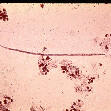The image is very small and difficult to discern, featuring a predominantly pink background with distinct visual details. At the top, there is a thin black border. A dark red line runs horizontally across the middle, exhibiting a slight incline towards the left. The image is peppered with dark burgundy red splatters, particularly concentrated towards the bottom half beneath the central line. One of the more notable splatters is situated in the upper left corner. The overall appearance is reminiscent of red paint splotches on pink paper, with granular, almost cellular textures that suggest a microscopic view of red-tinted particles.